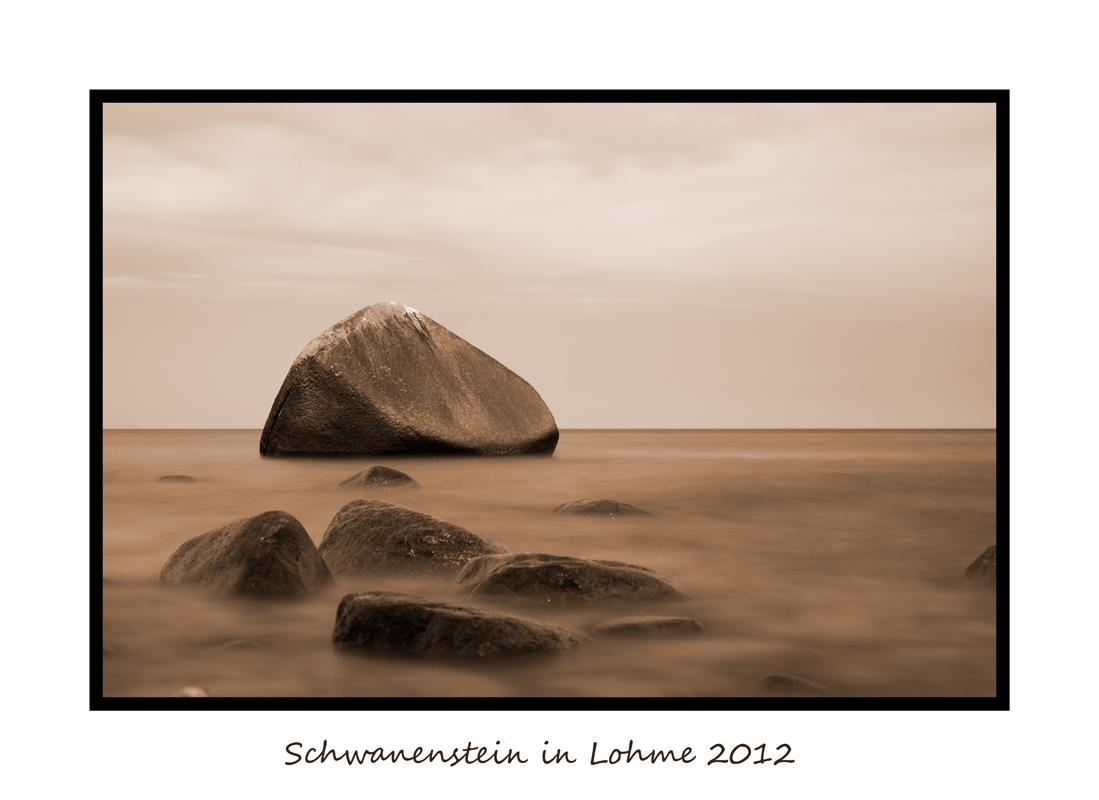The image titled "Swan Sting in Nome 2012" depicts a desolate desert landscape dominated by a muted brown color palette. The ground is a darker brown, dusty, and scattered with stones of various sizes. In the foreground, four medium-sized rocks of differing shapes stand prominently, surrounded by smaller stones barely poking out from the ground. In the distance, a very large, smooth stone with two visible surfaces and a cone-shaped top marks the far end of the scene. The sky above is a lighter brown mixed with hints of white, characterizing scattered clouds under an overcast, gray atmosphere. A brown line clearly separates the sky from the land. The entire image is encased in a black border with a cursive signature in black font at the bottom, marked with the year 2012. The air seems to be filled with a tan-colored fog that adds to the overall eerie and surreal ambiance of the barren desert landscape.